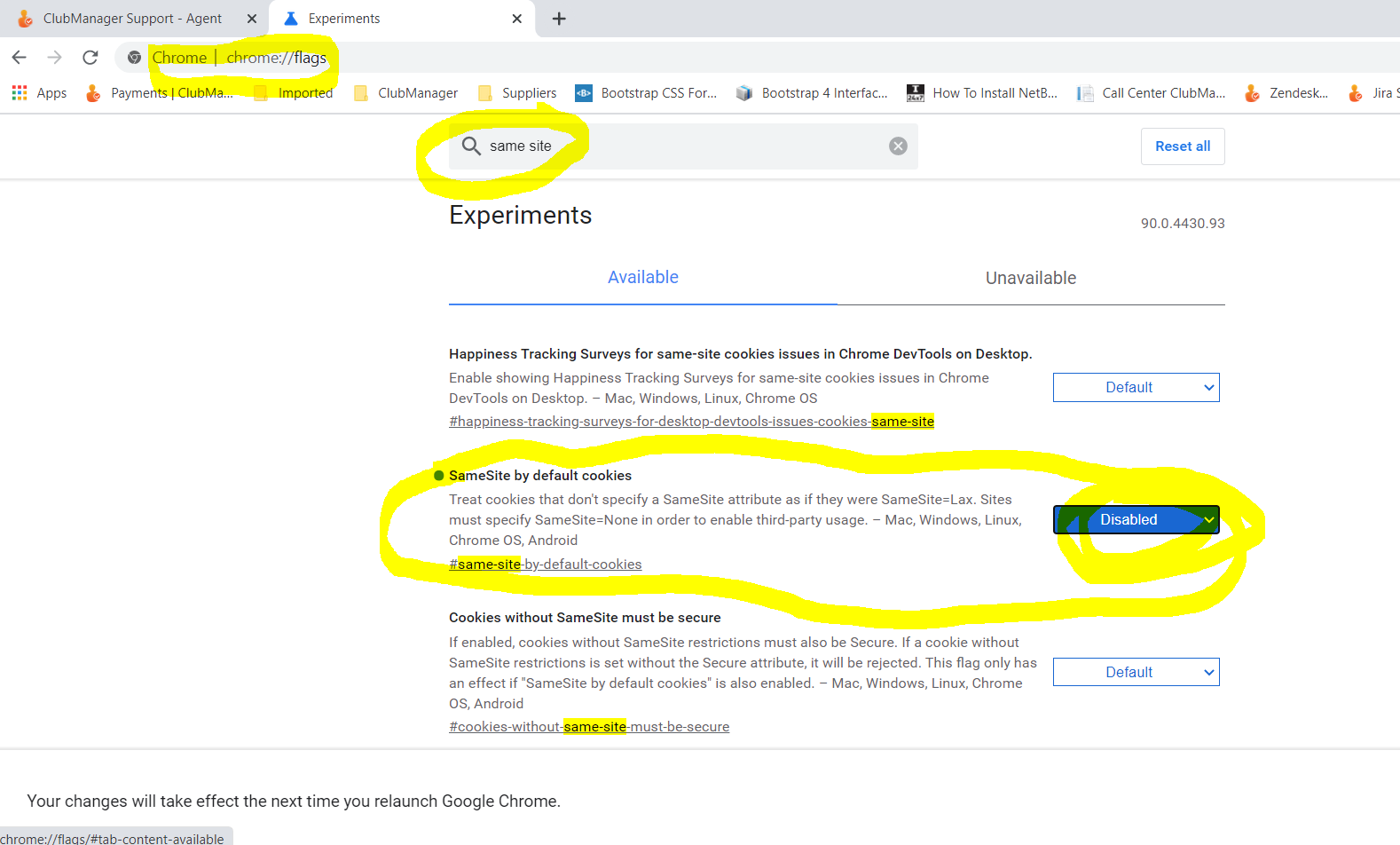Screenshot Description: This detailed screenshot captures the "Club Management Support Agent" interface displayed in the Chrome web browser. The entire page is emphasized with multiple yellow highlighter circles, targeting key sections of the interface. At the top, the title "Club Management Support Agent" is clearly visible, and the browser name "Chrome" is also highlighted.

Highlighted Sections:
1. "Same Site" is prominently circled in yellow marker multiple times, indicating its importance.
2. The "Experiments" section is visible, focusing on "Available" experiments, which is underlined in blue and contrasted with the "Unavailable" section marked in black.

Key Features:
- The "Happiness Tracking Surveys for Same Site Cookies Issues in Chrome Development Tools on Desktop" setting is featured, revealing instructions to enable this feature to track user happiness concerning same site cookies.
- Supported platforms for this feature include Mac, Windows, Linux, Chrome OS, and Android. This section is marked with hashtags for easy reference: #happiness-tracking-surveys-for-desktop-development, #tools-issues-cookies-same-site.

Additional Information:
- "Same Site by Default Cookies" is another significant focus. The description explains how cookies should be treated: cookies that don't specify a same site attribute will be treated as if they were Same Site=Lax, and sites must specify Same Site=none to enable third-party usage. Supported platforms again include Mac, Windows, Linux, Chrome OS, and Android, with specific hashtags: #same-site-by-default-cookies, #same-site.
- Highlighted in yellow is the explanation that cookies without a Same Site attribute must be secure. This security measure will reject cookies set without the Secure attribute unless the "Same Site by Default Cookies" is enabled, applicable on the same range of platforms.

The entire content within the screenshot is bordered by a yellow marker to encapsulate the focus areas. This screenshot serves as a detailed visual aid for understanding the configuration and implications of Same Site cookies within Chrome's development tools.